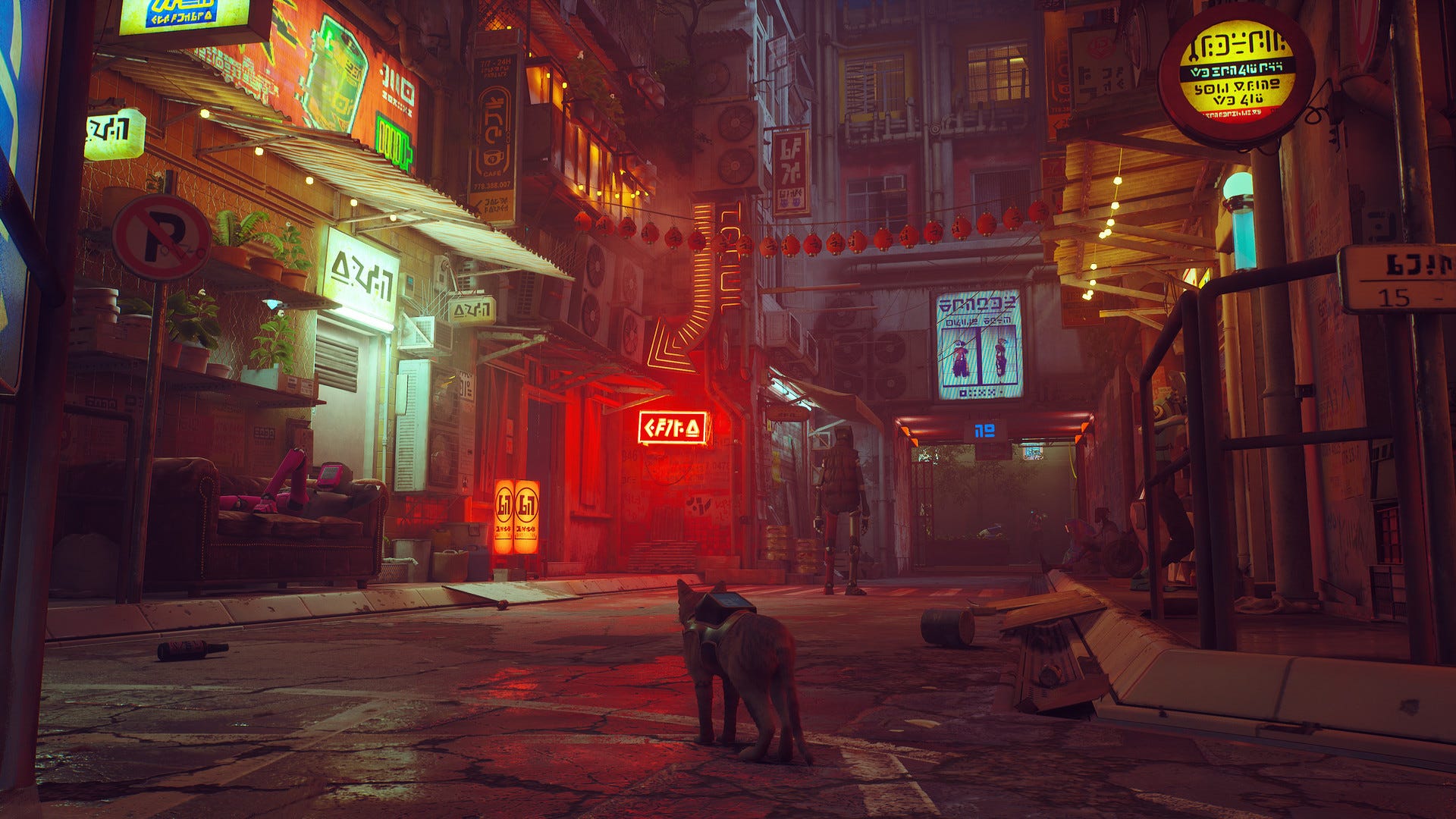The screenshot from the PS5 video game "Stray" captures a dark, futuristic alleyway, reminiscent of an Asian city street. The scene is illuminated by the red glow of neon signs and strung with Chinese lanterns, casting an evening ambiance over the setting. In the foreground, there is a cat with a small backpack walking through the street. Off in the distance, slightly blurred, is a tall, skinny robot. The alleyway is lined with various stalls and businesses adorned with symbols or Asian writing that suggest shops or other commercial establishments, although their exact nature is unclear. A sofa with a person in pink is visible in front of one shop, contributing to the rundown, almost dystopian feel of the scene. The overall mood is dark and somewhat gloomy, evoking a sleazy, late-night atmosphere.